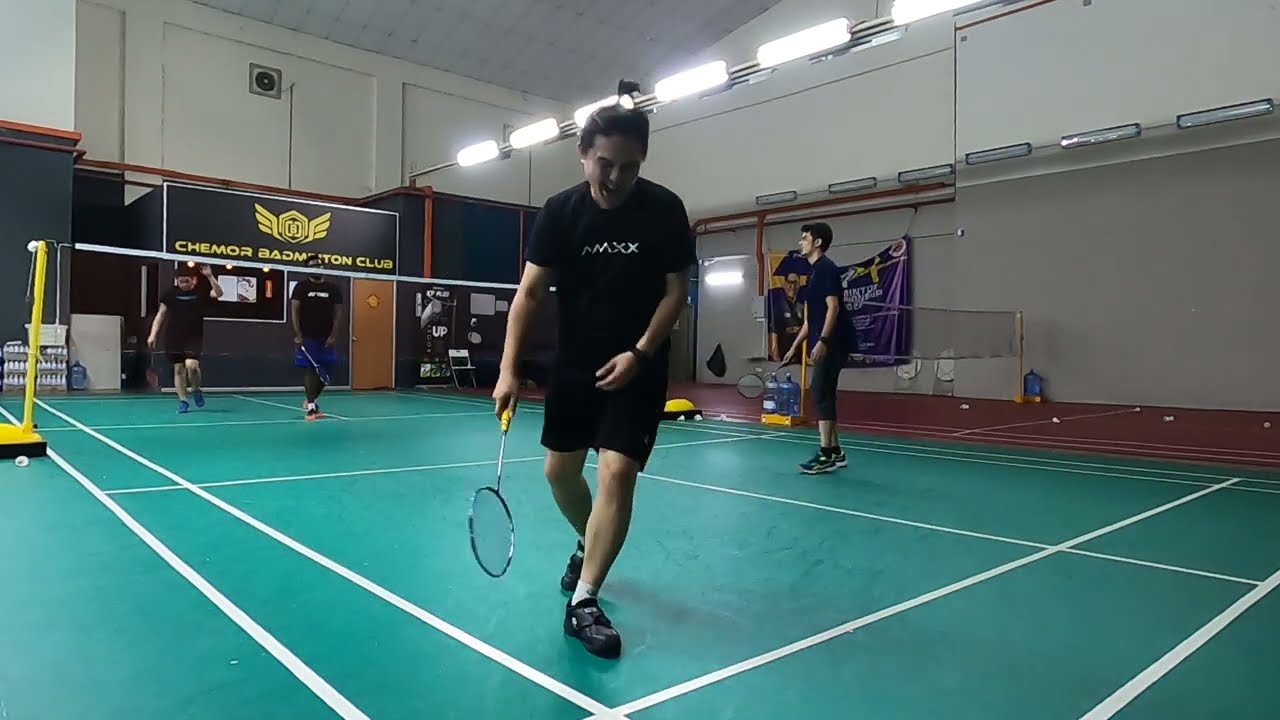In an indoor badminton court within a gymnasium characterized by very tall ceilings and bright fluorescent lights, a man stands at the forefront, facing the camera. He has dark hair and is dressed in a black shirt with white lettering, black shorts, black shoes, and white socks. He holds a badminton racket in his hand. The gym’s walls are an off-white color, and the floor is a bright tealish green with white stripes delineating the badminton court lines. Behind him, another player also holding a badminton racket, looks towards the opposite side of the net where their opponents are engaged in the game. On the far side, a sign reads "CHEMOR BADMINTON CLUB" with a logo above it. The scene captures the active moment of the game, highlighting the players' focused demeanor and the vibrant setting of the gymnasium.